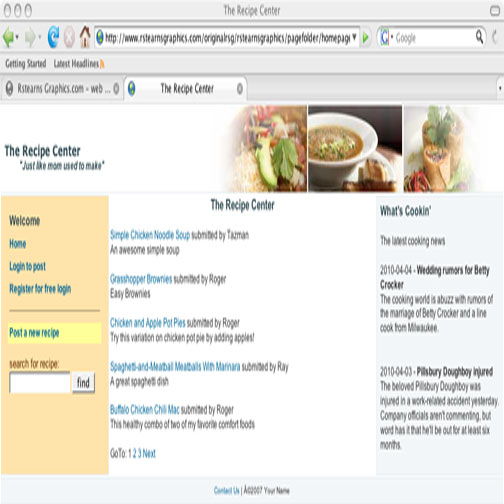A blurry image showcasing an old-fashioned web browser, possibly an early version of Mozilla, features a search bar and familiar navigation icons— a green back arrow and blue reload arrow. The title bar indicates the page belongs to "The Retcon Center" with the URL www.thumpingpig.com. The page headlines "Getting Started" beneath a gray navigation bar and displays two open tabs: "The Rector Diet Center" and "The Recipe Center". Prominent text reads "Just Like Mom Used to Make" beside a picture of a bowl of soup flanked by vegetables.

The section "The Recipe Center" highlights an array of links in blue, showcasing various recipes submitted by users. Among them are:
- Simple Chicken Noodle Soup by Tasman: An awesome simple soup.
- Grasshopper Brownies by Roger: Easy brownies (with a curious note questioning if they contain actual grasshoppers).
- Chicken and Apple Pot Pie by Roger: A variation of chicken pot pie with apples.
- Spaghetti and Meatballs by Ray: A great spaghetti dish.
- Buffalo Chicken Chili Mac by Roger: A healthy combo of comfort foods.

On the left-hand sidebar, links read:
- Welcome Home
- Log in to Post
- Register for Pre-login
- Post Recipe
- Search for Recipe with Search Box 

The right-hand sidebar titled "What's Cooking?" displays the latest cooking news dated 2010-04-04, mentioning wedding rumors related to Betty Crocker and a nameless cook, as well as an injury to the Pillsbury Doughboy that will sideline him for six months. The details remain blurry, adding to the nostalgic charm of this vintage website snapshot.